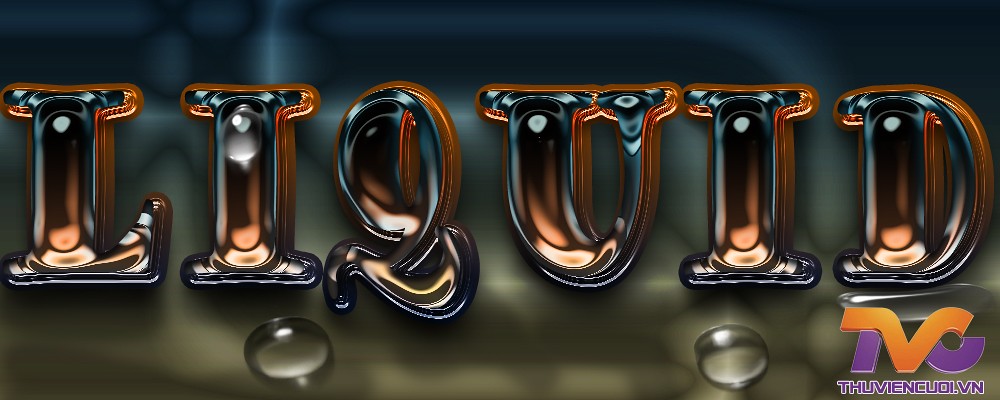The image is a computer-generated artwork, wider than it is tall, featuring the word "LIQUID" prominently in the foreground. The typography of "LIQUID" spans from the left to the right side of the image in all capital letters, characterized by a fluid, shiny, and metallic appearance, giving the letters a liquid-like texture. There are small water droplets beneath some of the letters, enhancing the illusion of liquidity. Reflections in shades of orange, gold, and white accentuate the liquid effect on each letter. The background is blurred, comprising mottled dark grays, very dark blues, and hints of greens, creating a stark contrast with the bright, glossy foreground. In the lower right-hand corner, there is an orange and purple logo consisting of intertwined letters that resemble "TVC" or "VIC," accompanied by an indecipherable foreign word underneath it in a similar color scheme. The overall style blends elements of illustration and graphic design.